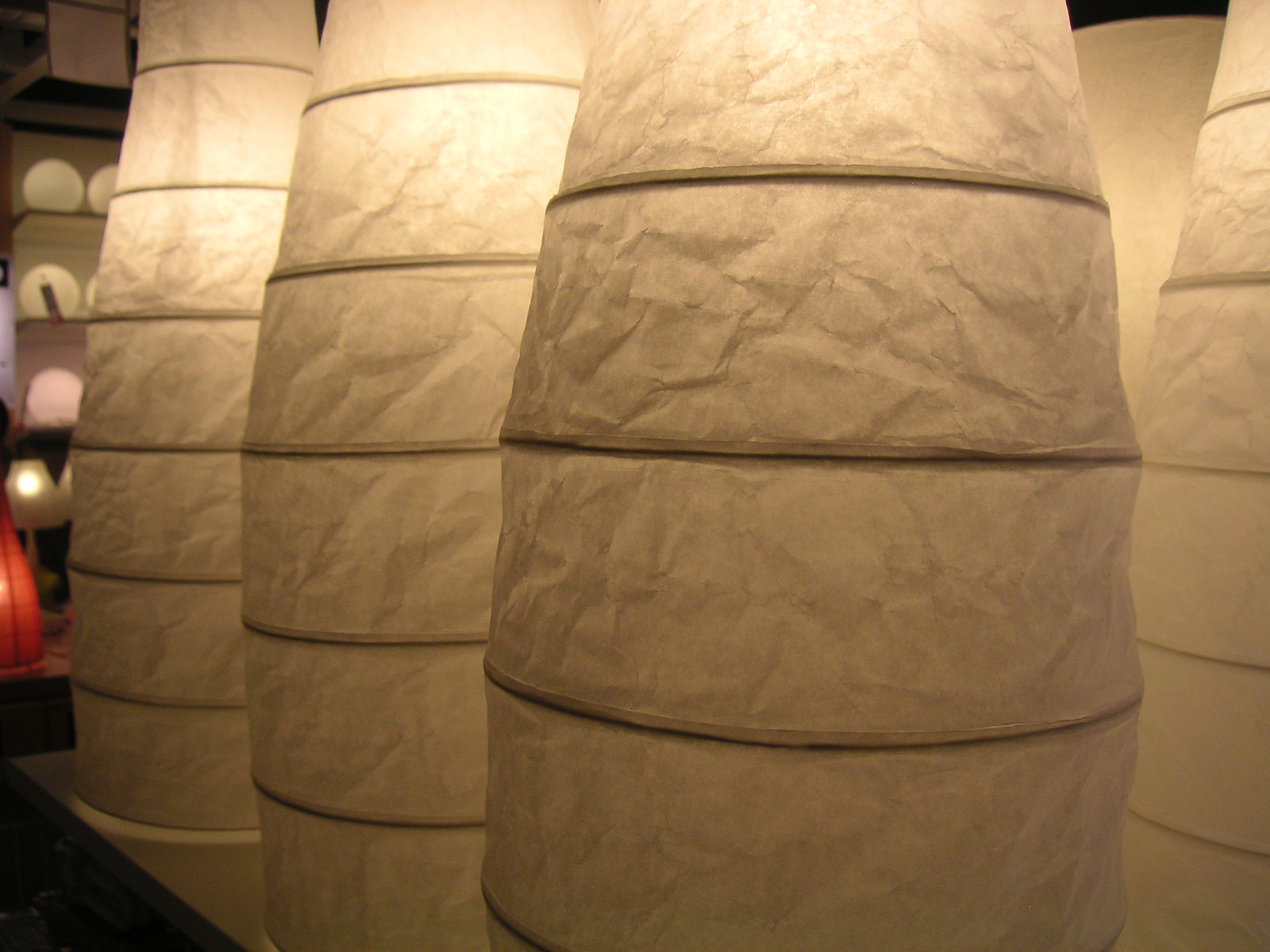The image is a close-up photo showcasing an arrangement of several tall, cylindrical white lampshades or paper lanterns, tapering slightly towards the top. Each lamp features a warmly lit interior, creating a cozy glow that emanates from within. These lamps have a distinctive tiered design with equidistant bands encircling them, resembling segmented sections akin to an upright maggot or grub. The primary focus reveals three lamps lined in a row, with a hint of additional lamps peeking from a second row behind. They appear to be crafted from a material similar to thin white paper, with reinforcing seams demarcating each tier. The setting is suggestive of a home goods store, as shelves stocked with plates and a variety of other lighting features, including some possible additional colors such as pink or red, are visible in the blurred background.